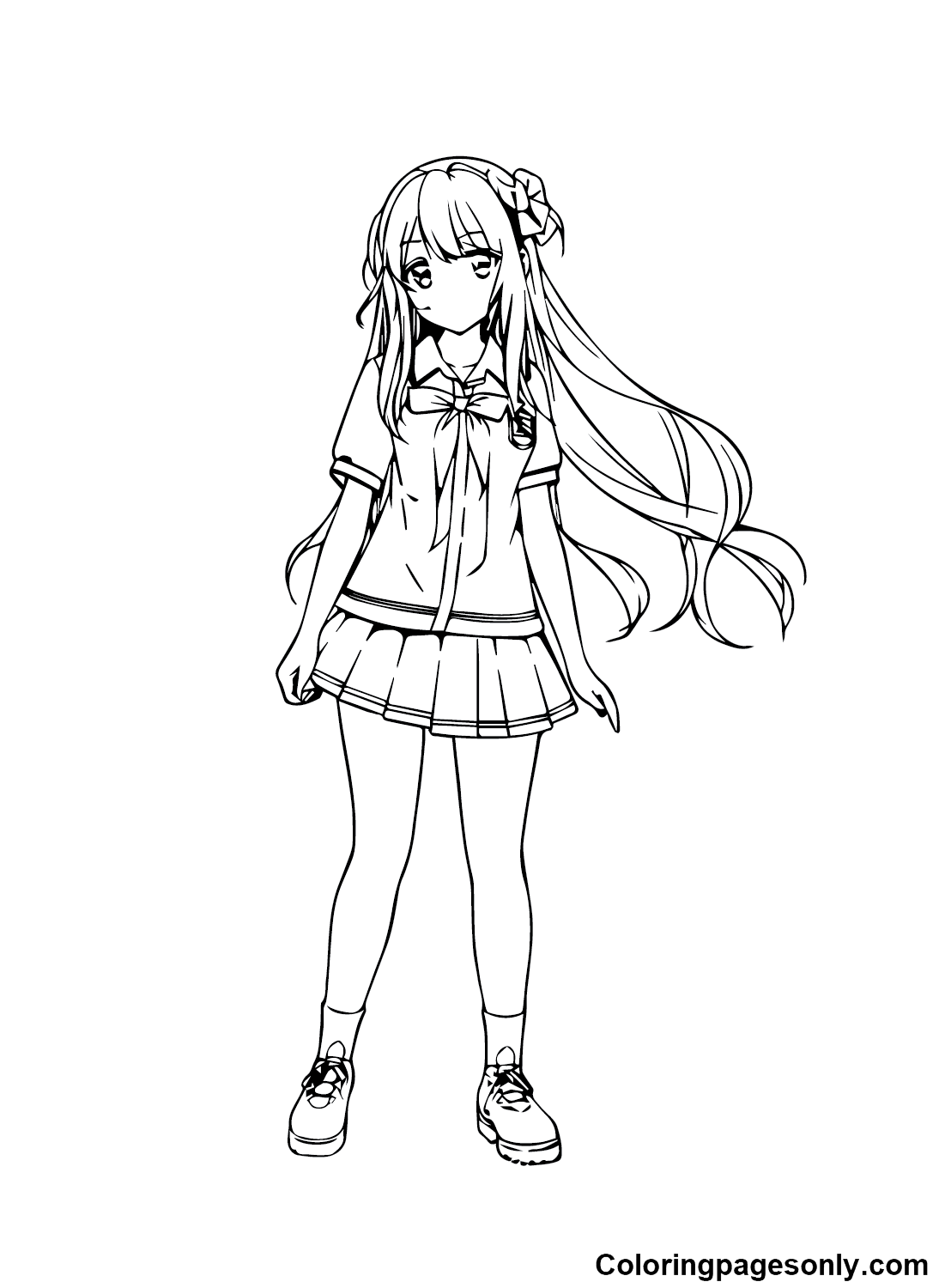The image portrays an anime-style, black and white line drawing of a girl, resembling a page from a coloring book. She stands vertically in the center of the drawing, which has no border and is set against a plain white background. The only text appears in the lower right corner, stating "coloringpagesonly.com."

The girl is wearing a typical schoolgirl uniform that features a short, pleated skirt and a short-sleeved blouse. The blouse is detailed with buttons down the front and a bowtie ribbon at the collar, along with a badge, suggesting she might belong to a private school. She has long, wavy hair that falls to her hips, with bangs framing her face. A ribbon is tied in her hair, adding to her schoolgirl appearance. 

Her facial features include large, expressive eyes, but her nose and mouth are not depicted. She is shown with bare legs, wearing white socks paired with low-cut shoes that resemble hiking boots with visible shoelaces. The girl's straight, relaxed posture—with her hands resting at her sides—conveys a calm and approachable demeanor, ready to be brought to life with color by a child.